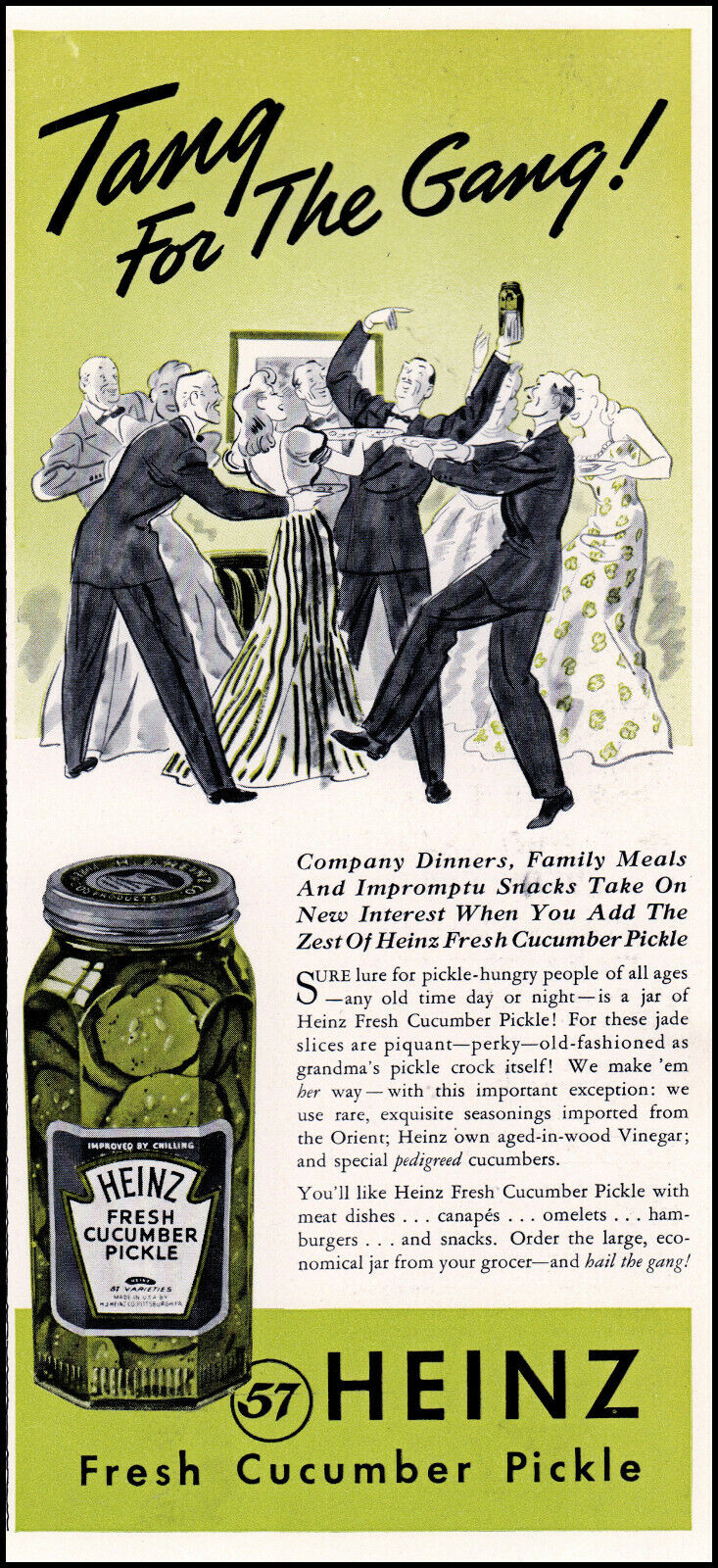This image depicts a vintage magazine advertisement for Heinz Fresh Cucumber Pickle, framed with a black border. The advertisement features a festive scene at the top where elegantly dressed men in tuxedos and women in long gowns are joyfully dancing in a room adorned with a mirror reflecting the lively party. The backdrop is a light green wall, and the dancers hold jars of pickles, enhancing the celebratory atmosphere.

Below the image of the party, a detailed description highlights the versatility and appeal of Heinz Fresh Cucumber Pickle, encouraging its use at company dinners, family meals, and impromptu snacks to add zest. The text promotes the pickles as suitable for a variety of occasions and dishes, noting the unique seasonings and high-quality cucumbers used in their production.

In the bottom left corner, prominently displayed, is the product itself—a glass jar with a steel cap, labeled “Heinz Fresh Cucumber Pickle.” The jar shows off the crisp green pickle slices inside. Finally, at the bottom of the ad, a green rectangular strip features the iconic Heinz logo with the number "57" in a circle followed by the product name "Heinz Fresh Cucumber Pickle," completing the nostalgic and enticing appeal of this vintage advertisement.